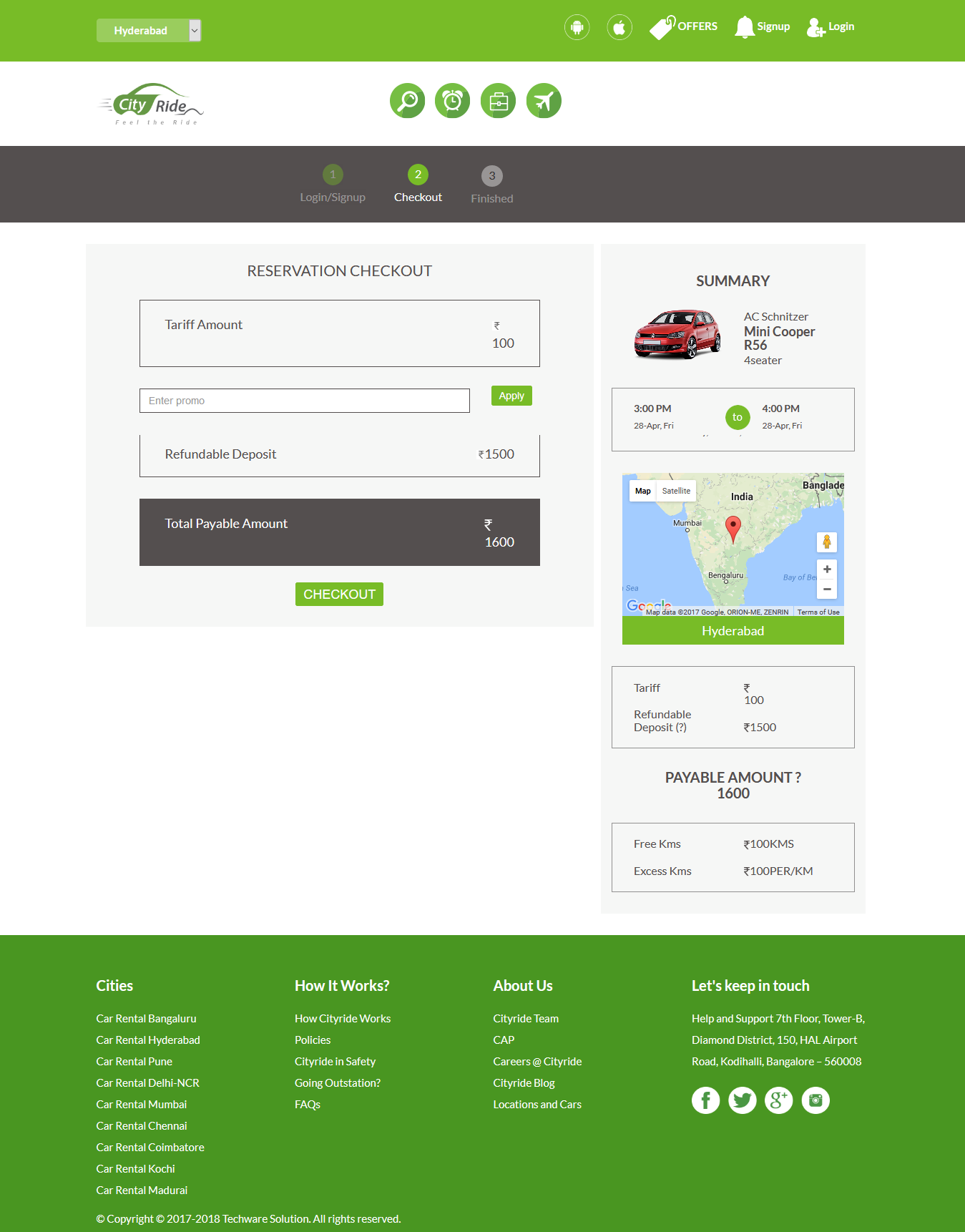The image appears to be a website interface for a car rental service named "City Ride." The website features a clean layout with various interactive elements and information.

At the top-left corner, there is a green strip with a drop-down menu labeled "Hyderabad." Adjacent to it are circular icons representing Android and Apple applications, followed by options for "Offers," "Sign Up," and "Log In."

The centerpiece of the header showcases the "City Ride" logo, which has a stylized car motif. The "City" part of the logo is white and set against a green background resembling the front part of a car, while "Ride" is black, designed to look like the back wheel of the car.

Below the logo, there are circular buttons for different functionalities: search, alarm, clock, suitcase, and an airplane icon. 

The section beneath this has a slate gray strip featuring a three-step navigation process: 
1. Sign In / Log In / Sign Up 
2. Check Out 
3. Finish

The current step highlighted is "Check Out." This part provides details such as "Reservation," "Tariff Amount: 100 INR," and an option to enter a promo code with a green "Apply" button next to it. There is also information about a "Refundable Deposit: 1500 INR" and the "Total Payable Amount: 1600 INR." At the bottom, there is a green "Check Out" button to proceed with the payment.

The overall design is user-friendly, guiding users through the car rental process with clarity.